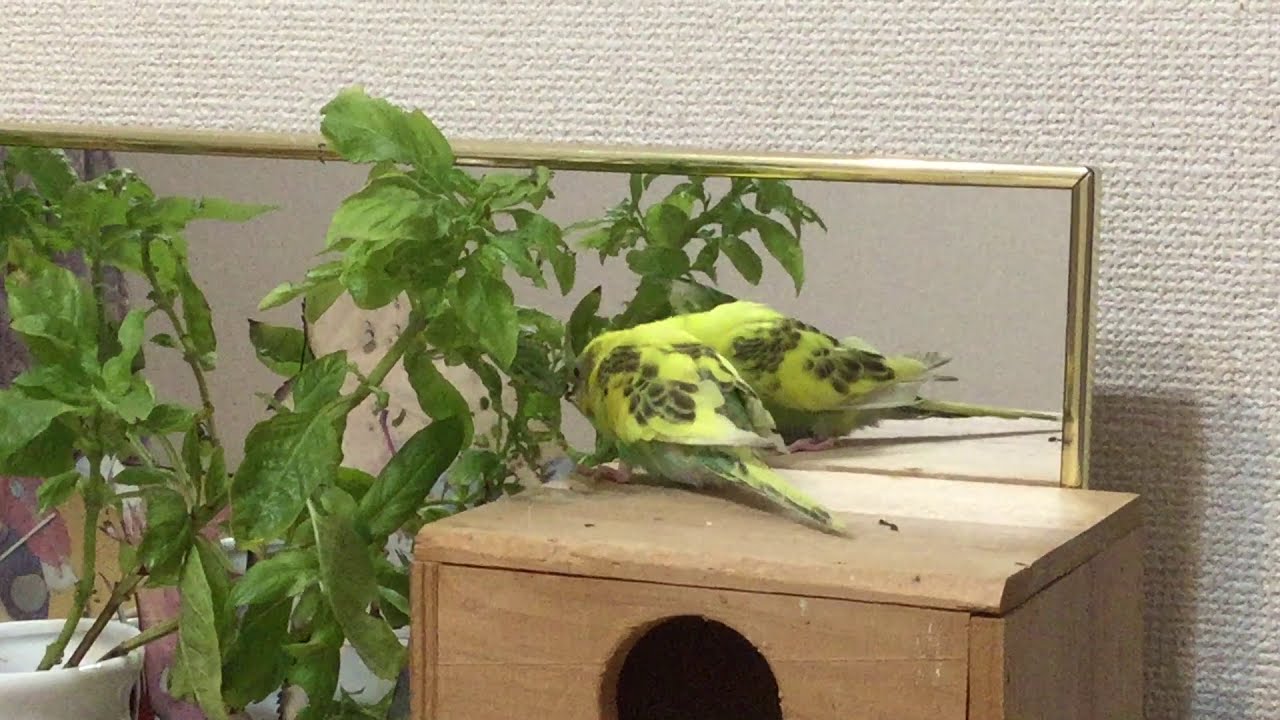The image depicts a vibrant yellow parakeet with black spots on its wings and hints of green, resembling the color of Mountain Dew. The bird is perched on a wooden object that serves as both a small desk and a home, characterized by a circular opening in its front. This wooden piece is placed near a large, elegant mirror with a gold or brass frame, which extends across the wall and captures the reflection of the bird and surrounding objects. To the left, a white vase holds green plants with several branches extending in various directions, contributing to the serene and laid-back atmosphere of the room. The mirror’s reflection enhances the brightness and calmness of the space, making it an inviting and aesthetically pleasing setting. The wall behind is unique, possibly made of textured stucco, adding a distinctive touch to the room's overall decor.